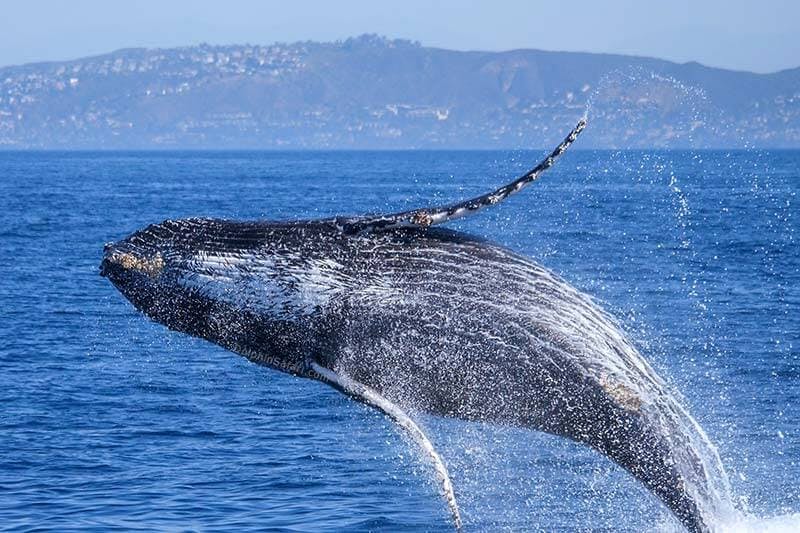This rectangular image captures a dramatic scene of a whale, likely a humpback, breaching out of the ocean. The whale's large body arches sideways, with its dark gray back and white underbelly clearly visible. Water splashes surround the whale as it propels itself out of the vibrant blue sea, creating an energetic display. The whale's pectoral fins stretch outward, adding to the sense of motion. Its tail remains partially submerged, hidden beneath the water and the photo frame. The image's background features a faded, hazy sky and a distant hillside adorned with houses, trees, and natural terrain, all bathed in a subdued grayish-blue light. The main focus remains on the majestic whale, which stretches horizontally across the frame, exuding power and grace.